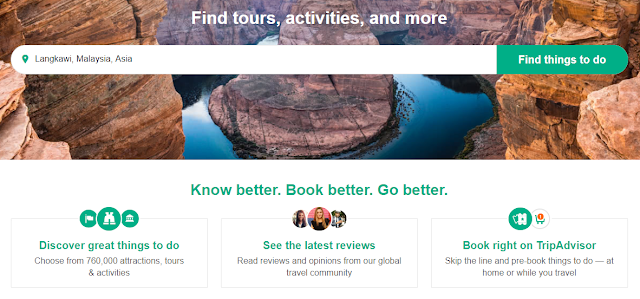A screenshot of the TripAdvisor website features a dual-section layout. The background showcases a picturesque, yet indistinct, scene potentially located in Asia, characterized by rocky cliffs surrounded by water. The landscape, though realistic, is not immediately recognizable. Overlaid in the foreground, white text reads, "Find tours, activities, and more," accompanied by a search bar filled with an Asian location name, culminating in a "Find things to do" button on the right.

Below this image, TripAdvisor's slogan, "Know better, book better, go better," is prominently displayed. The section is divided into three informational blocks. On the left, "Discover great things to do" highlights TripAdvisor's extensive offerings with, "Choose from 760,000 attractions, tours, and activities," emphasized by green icons. The center block, "See the latest reviews," is similarly accented with person-like icons, directing users to explore recent visitor feedback. The rightmost block, "Book right on TripAdvisor," completes the trio with more details about the site's booking capabilities, each section marked by icons featuring the TripAdvisor logo.